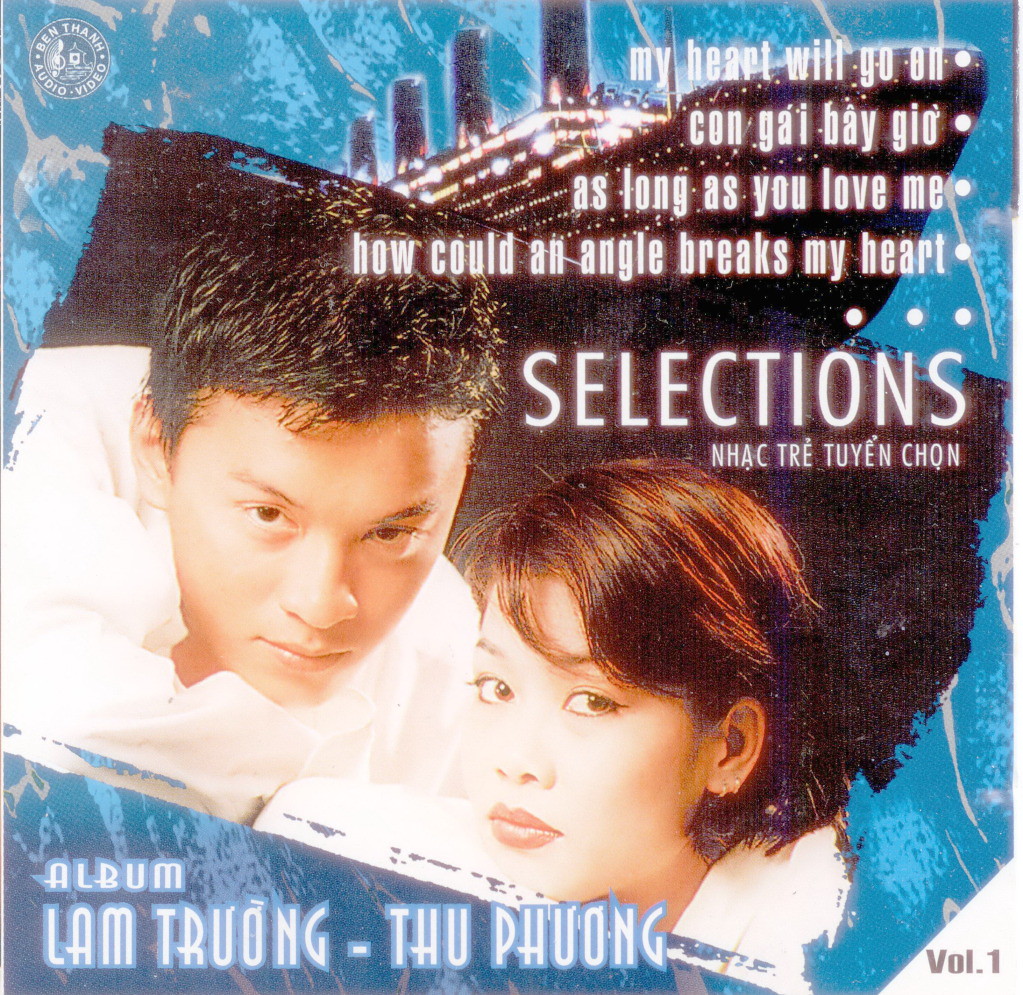The album cover features a blue abstract background with splashes of gray and bears several significant details. At the top left-hand side, a circle with a musical note contains the text "Ben Fan Audio Video." Moving towards the center, an outline of the Titanic with all its lights on is prominently depicted. Just beneath the ship, there is a photograph of a man and woman both dressed in white, suggesting they are likely the singers of the album. 

In the top right-hand corner, the album lists its featured tracks in white text, including "My Heart Will Go On," "Kon Gai Bei Go," "As Long As You Love Me," and "How Can an Angel Breaks My Heart." Below this, the album title "Selections" alongside "Nak Trey Tiyan Chan" is visible. At the bottom, specifically on the left-hand side, "Album" along with the names "Lam Truong" and "Thu Phuong" can be found, and on the bottom right side, it states "Volume 1."